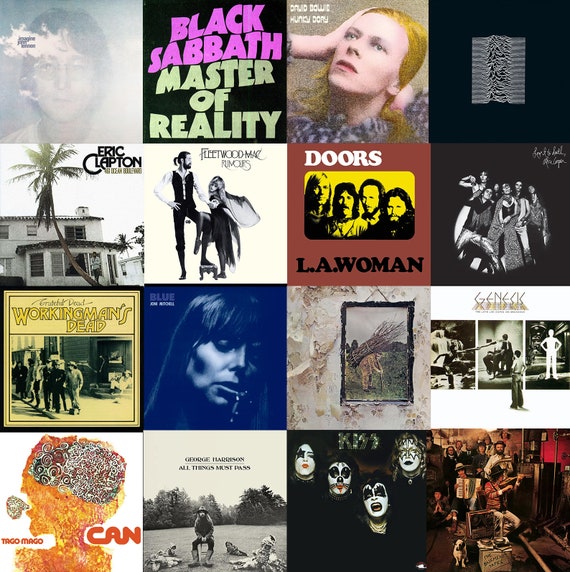This composite montage features 16 classic rock album covers arranged in a 4x4 grid, showcasing an iconic collection. In the top left, John Lennon’s "Imagine" album features Lennon himself, wearing large glasses and a white t-shirt on a grayish background. Adjacent to this is Black Sabbath's "Master of Reality" in its bold, dark typography. Next is David Bowie's "Hunky Dory," illustrating a young Bowie with reddish blonde hair in a colorized photo. Completing the top row is an album cover displaying a sonogram-like graph on a black background, more abstract and unidentifiable.

The second row begins with an Eric Clapton album, depicting a single palm tree in front of a Californian house facade. Following this is Fleetwood Mac's "Rumors," renowned for its stark imagery. The Doors' "L.A. Woman" is next, featuring a photograph of the band members set within a distinctive yellow rectangle on a brown background. The final image in this row is currently undiscernible.

The third row starts with Grateful Dead’s "Workingman’s Dead," characterized by a black and white photo of them. Joni Mitchell's "Blue" follows, marked by the dark blue cover and her portrait. Led Zeppelin's untitled album, commonly referred to as "Led Zeppelin IV," presents an old man with a heavy sack of kindling against a stony backdrop. Next is an album by Genesis, exhibiting a typically intricate cover design.

The final row features "Tago Mago" by Can, known for its distinctive and experimental style. George Harrison’s "All Things Must Pass" comes next, portraying Harrison seated contemplatively. A Kiss album cover follows, showing the four members in their iconic makeup. The last album in the montage is more ambiguous, possibly a painted cover showing band members including an accordion player and a dog, giving it a vintage artistic flair.